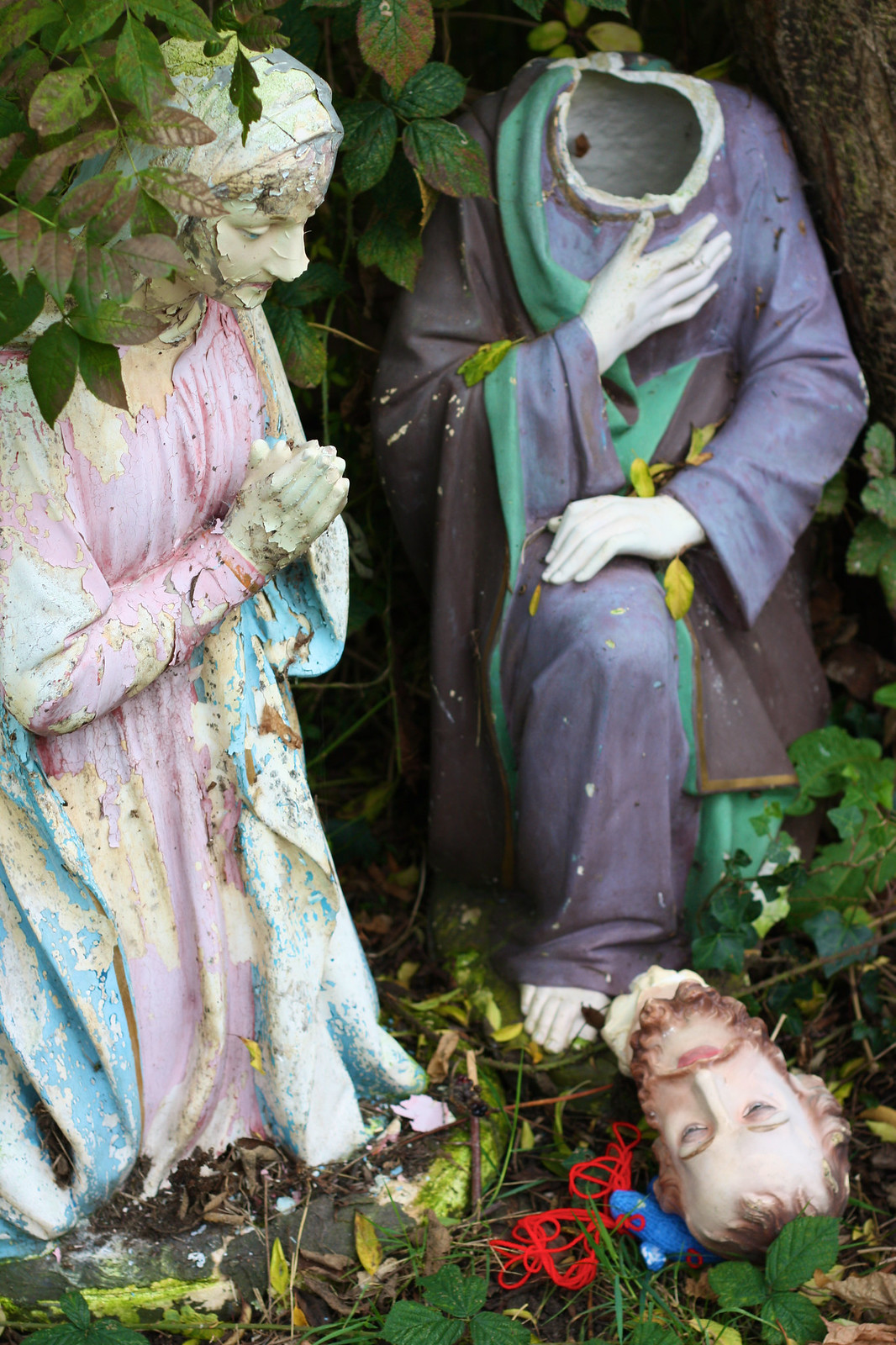In this image, we observe two religious statues in a garden, both surrounded by lush green leaves and overgrown plants, indicating a sense of abandonment. On the left stands a statue of a woman, her head covered and her hands clasped to her chest as if in prayer. She is adorned in a pink dress with a blue shawl, though the paint is noticeably peeling. To her right is a statue of a man, kneeling in a blue-grey robe with green and black accents. Uniquely, this statue's head is missing from the torso and lies detached on the ground, positioned against some green leaves and accompanied by what appears to be a blue stuffed animal with a red cord. The man's exposed toes are visible as he wears no footwear. Above them, a tree branch dangles, partially captured with its bark and leaves drifting into the frame. The disarray and the decapitated statue evoke a mysterious and somewhat eerie ambiance, intensified by the face of the male head, which strikingly resembles Jesus.